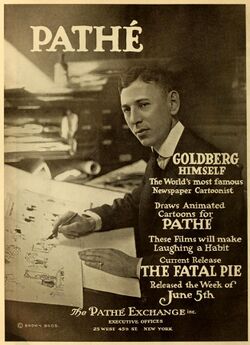The image is a sepia-toned black and white photograph that appears to be the cover of a vintage magazine or newspaper from the 1920s or 1930s. Centered in the composition, a man with short-cropped hair, dressed in a suit with a tie and a rounded-collared shirt, faces the camera while slightly turning his head to the side. He is engaged in drawing at a large easel, his right hand holding a pen over a sheet of paper filled with sketches, while his left hand rests on a blank sheet beneath it. The background features bookcases and shelves stacked with papers, indicating his workspace.

Prominently displayed on the cover, in white letters, is the title "Pathé," with an accent over the "E." Accompanying text on the left side identifies the man as Goldberg, famously known as the world's most celebrated newspaper cartoonist. The cover announces that Goldberg draws animated cartoons for Pathé, promising that these films will make "laughing a habit." It highlights a specific release, "The Fatal Pie," scheduled for release the week of June 5th. At the bottom, partially obscured text reads "The Pathé Exchange." The overall design and elements suggest this is a promotional cover dedicated to a significant figure in animation and cartooning.